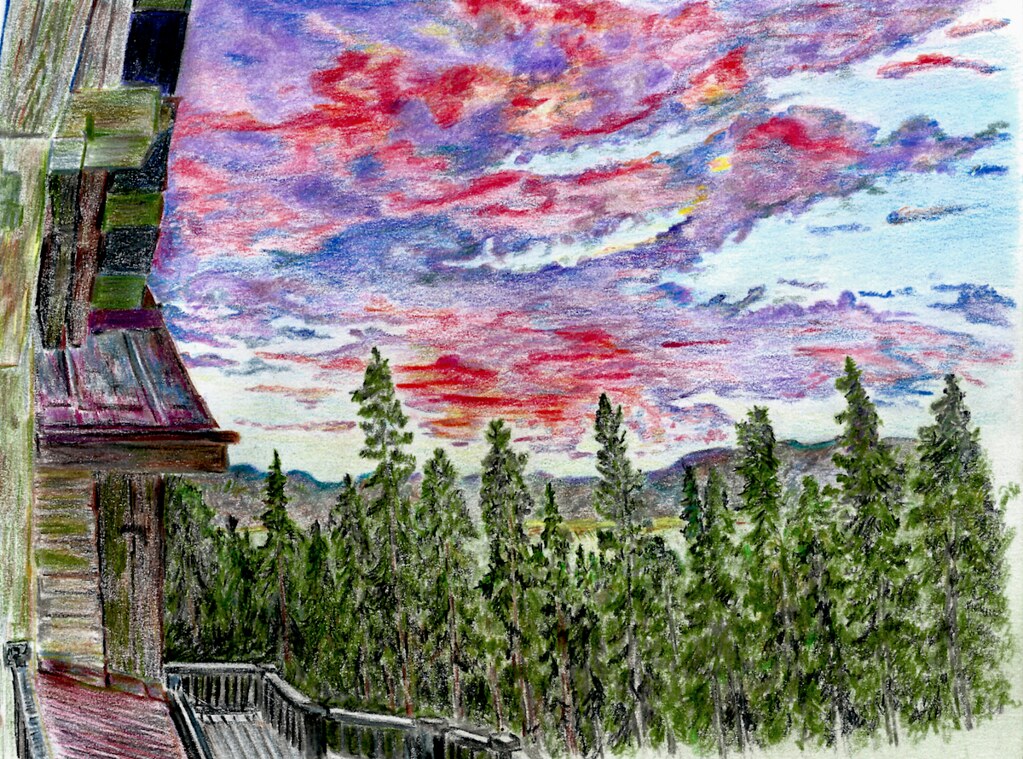The painting, possibly crafted with pastels, depicts a serene and captivating landscape. The sky, a mesmerizing blend of sky blue, is dominated by clouds lit from underneath, showcasing stunning hues of purple, red, and dark blue. On the left side of the artwork, a portion of a log cabin or lodge is visible, characterized by its log construction and chinking, capped with a tin roof. This structure appears to be two stories high, with a deck featuring a handrail. Stretching from the lodge to the right edge of the illustration is a row of tall, narrow conifer trees. Beyond this natural barrier, a valley or field extends into the distance, framed by a majestic mountain range in the background. The overall effect of the painting is both enchanting and tranquil, capturing the beauty of the landscape with remarkable detail and depth.